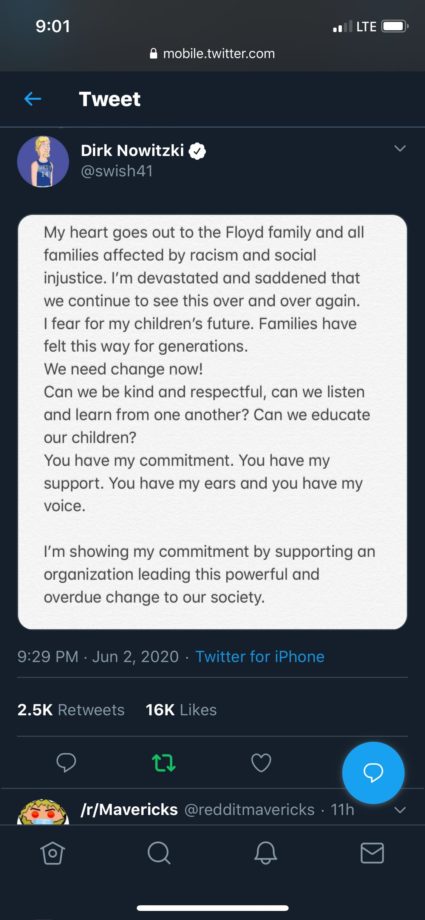**Detailed Caption:**

The image depicts a screenshot of the Twitter mobile interface displayed on an iPhone. At the top part of the screen, the URL "mobile.twitter.com" can be seen, indicating that the Twitter app for mobile is open. On the left-hand side of the screen, the word "Tweet" is visible alongside the user's profile name, "Dec Nowitzki."

The Tweet itself expresses sorrow and a call for action against racism and social injustice. The text, written in black, reads: "My heart goes out to the Floyd family and all families affected by racism and social injustice. I am devastated and certain that we continue to see this over and over again. I fear for my children's future. Families have felt this way for generations. We need change now. Can we be kind and respectful? Can we listen and learn from one another? Can we educate our children? You have my commitment. You have my support. You have my ears and you have my voice. I am showing my commitment by supporting an organization leading this powerful and overdue change to our society."

The Tweet was posted at 9:29 PM on June 2, 2020, via Twitter for iPhone. There are engagement metrics visible below the text: 2.5k retweets, 16k likes, with the retweet icon highlighted in green indicating the user has also retweeted it. Additionally, there is a heart icon for likes. At the bottom right of the screen, there is a blue button for messaging.